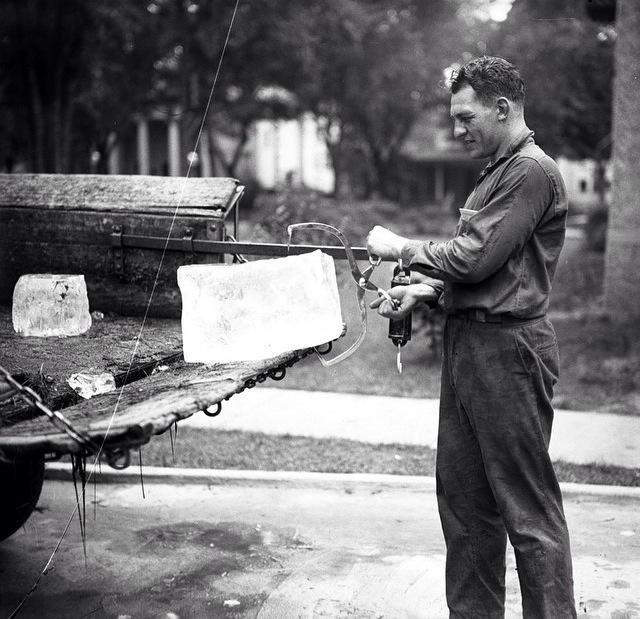This black-and-white photograph captures a moment from what appears to be the 1940s. A man with short dark hair, dressed in blue jeans and a dark long-sleeved shirt, is clean-shaven and has a small, satisfied smile on his face. He stands beside an old, well-used truck, its bed down and held by chains, revealing a dirty surface. The man uses a pair of metal ice tongs to lift a large, rectangular block of ice from the truck’s bed. Another, smaller, cube-shaped block of ice sits toward the back of the truck, which is flanked by wooden slat sides leaning precariously. In his hand, the ice tongs clamp onto the ice securely, resembling forceps or large clamps. The scene is set on a cement street with a blurred background featuring a sidewalk, several trees, and indistinct houses, suggesting a suburban neighborhood. A set of scales with a dangling hook is visible on the side of the truck, highlighting the utilitarian nature of the scene. The man's focused, yet content expression suggests he takes pride in his work, amidst this snapshot of post-war America.